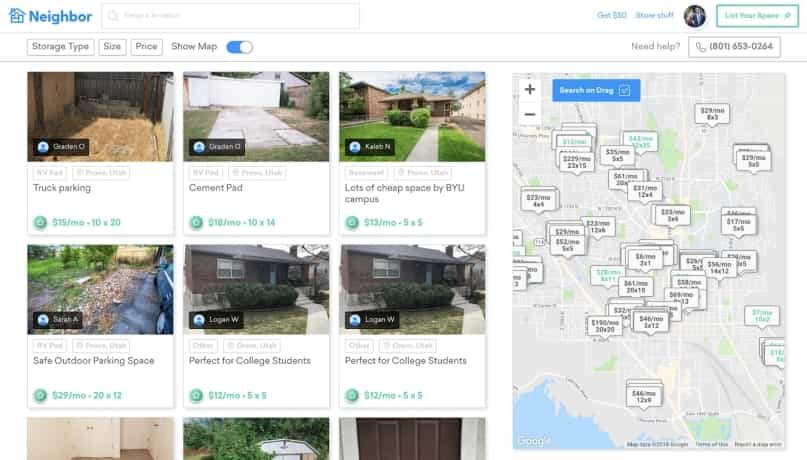Screenshot of the Neighbor website, capturing the user interface and several functional elements. At the top left, the Neighbor logo is prominently displayed in blue text. Adjacent to the logo, there's a search bar integrated into the header. Over on the top right side of the header, there’s a partially blurred section with the text likely reading "Get Stuff" and a small profile icon, indicating user account access.

Beneath the header, there are filter options that allow users to refine their search by storage type, size, and price. There's also a toggle button labeled "Show Map" which is currently enabled. On the far right below the header, a "Need Help" button and accompanying phone number are available for users requiring assistance.

The main content area features a variety of listings, each detailing different storage and parking options. Examples include "Truck Parking," "Cement Pad," and "Lots of Cheap Space by BYU Campus," all aimed at different storage needs. Several listings highlight suitability for college students, indicative of the target demographic, with prices such as $15 per month for a 10x20 truck parking space, denoted in green text.

On the right half of the screenshot, there’s a large interactive map displaying the locations of all the listed storage options. The map includes zoom in and zoom out functionalities, allowing users to explore the geographical distribution of available spaces.